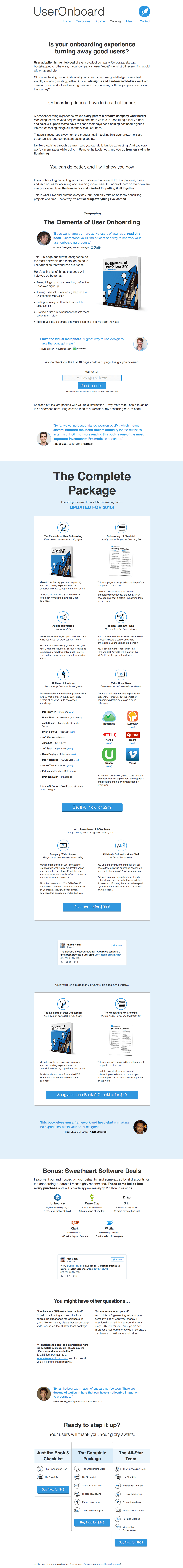The image showcases a webpage from a website named "User On Board" with both 'U' and 'O' capitalized. At the far right of the page, a logo is present, though the tiny print makes it unreadable. The page begins with a black title, followed by paragraphs of text that are also difficult to discern due to their small font size. 

In the lower-left section of the image, there is a graphic, labeled as page one, with another image situated directly below it. This suggests a multi-page view, possibly indicating various user options, but the small typeface again hampers readability.

At the bottom of the webpage, there is another section with black text at the top, followed by three progressively enlarging boxes. The content within these boxes is nearly illegible, though they are highlighted in blue, signaling their importance. Additionally, three blue bars appear at the bottom, with the central image outlined in a light blue box, further emphasizing its significance. Overall, while the website's specific details remain unclear due to the minuscule font, the layout hints at a structured presentation of user options.